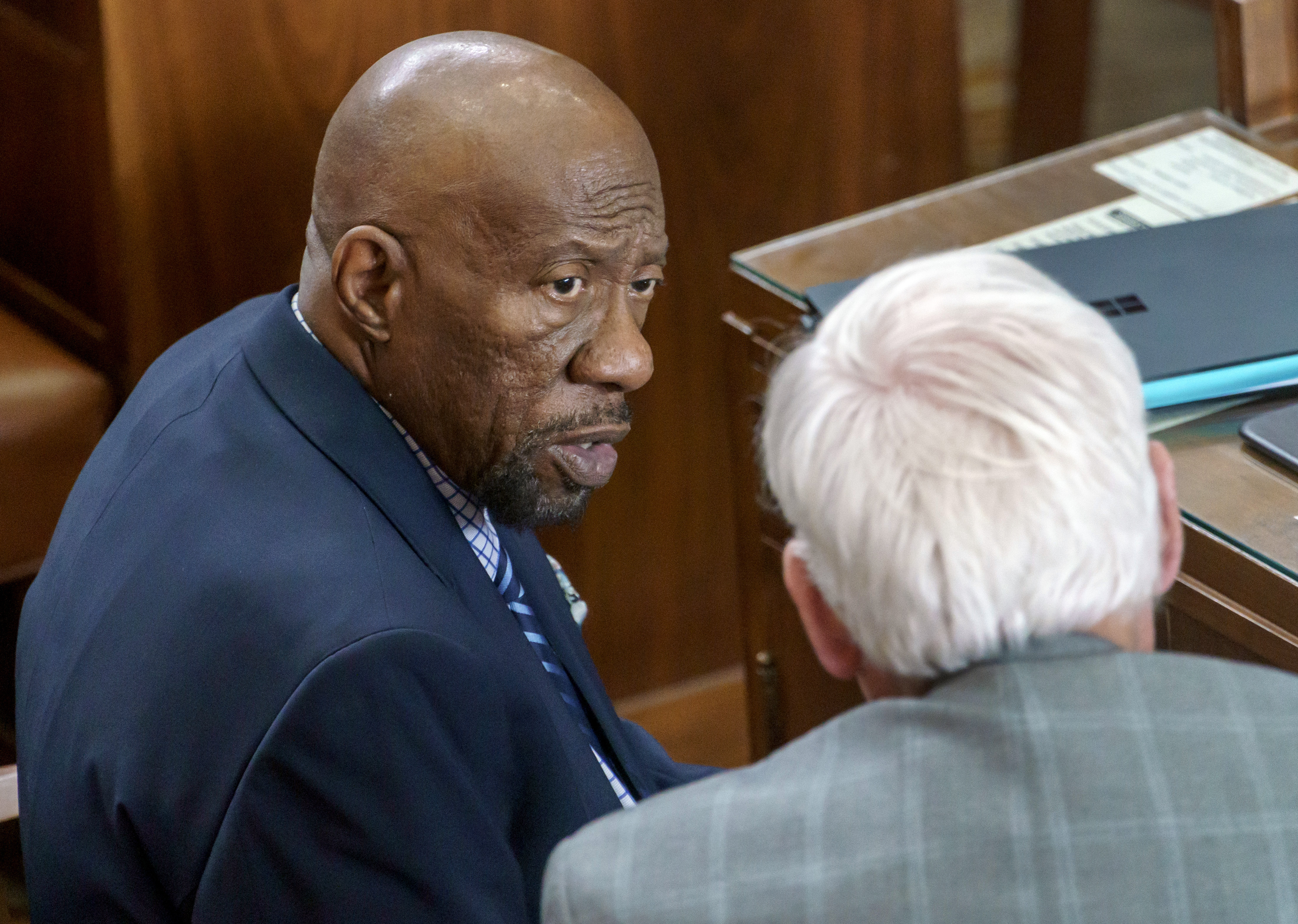This detailed photograph captures an intense moment between two men in an office or courtroom-like setting. On the left, an elderly African American man, entirely bald with a black mustache and partial beard, is dressed in a dark blue suit paired with a blue and white striped shirt and a matching blue and light blue striped tie. He gazes intently at another man whose profile is mostly obscured, save for his all-white hair, indicating his senior age. This second man dons a gray striped suit. The environment is richly adorned with wooden décor, giving it a solemn and official feel. In the background, a desk is scattered with various papers, folders, and what appears to be a black laptop or folder, reinforcing the seriousness of their interaction. The scene is immaculately lit, highlighting the concern evident in the African American man's face, suggesting they might be attorneys or investigators in deep discussion.